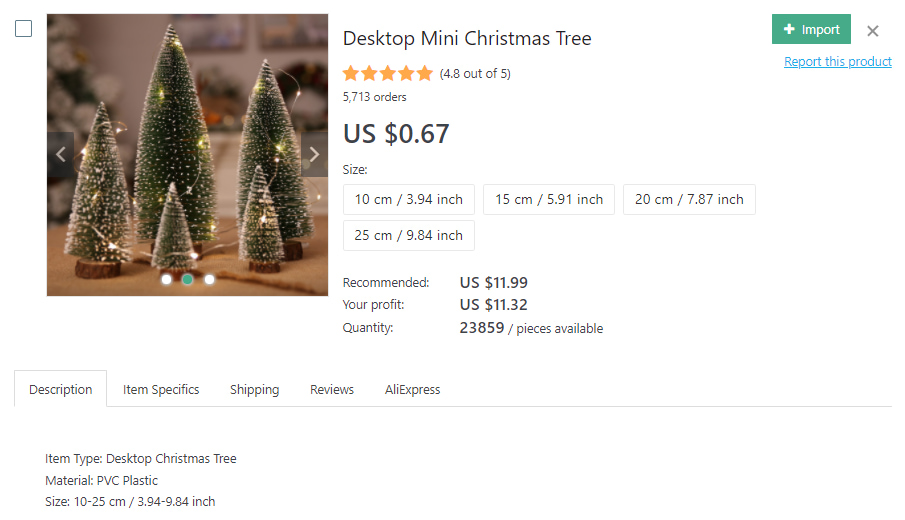**Screenshot of SOC Website: Detailed Description**

The screenshot captures a SOC website with a clean, all-white background. In the top left corner, there’s an outlined black square with a white interior. Centrally located within this square is an image measuring approximately three inches by three inches. The image depicts a gray, out-of-focus background with a few distinguishable elements. 

In the image's left corner, a small Christmas tree can be partially seen. In the foreground, there is a wooden table showcasing a variety of miniature Christmas trees. The table hosts a medium-sized toy Christmas tree from which a larger tree extends almost to the top of the image. Beside it, to the right, there are medium and small trees arranged in a descending height pattern, creating a visually appealing setup. 

On the right side of the image, bold black text reads, "Desktop Mini Tree." Adjacent to this, a green rectangle with a white plus sign features the text "Import" in white. To the right of this, there's a black "X" symbol. Below “Desktop Mini Tree” but on the left side, five yellow stars indicate a rating of 4.8 out of 5 based on 5,713 orders. 

Underneath this rating, the price is stated as "U.S. 67 cents." Further down, the section labeled "Size" offers three tabs laid out horizontally, each representing different sizes. Below these tabs, there's an additional size option listed to the left. 

The section titled "Recommended" follows suit, continuing to the right stating "U.S. 1,199." Subsequent information includes "Your Profit: 1,132" and "Quantity: 23,859 pieces available." 

Directly beneath the displayed trees, the word "Description" appears in black text, followed by sections for "Item Specifics," "Shipping," "Reviews," and "AliExpress" arranged horizontally. 

In the bottom left corner of the screen, there’s a list detailed by three lines of text:
- Item Type: Desktop Christmas Tree
- Material: PVC Plastic
- Size: 10 to 25 centimeters / 3.94 to 9.84 inches.